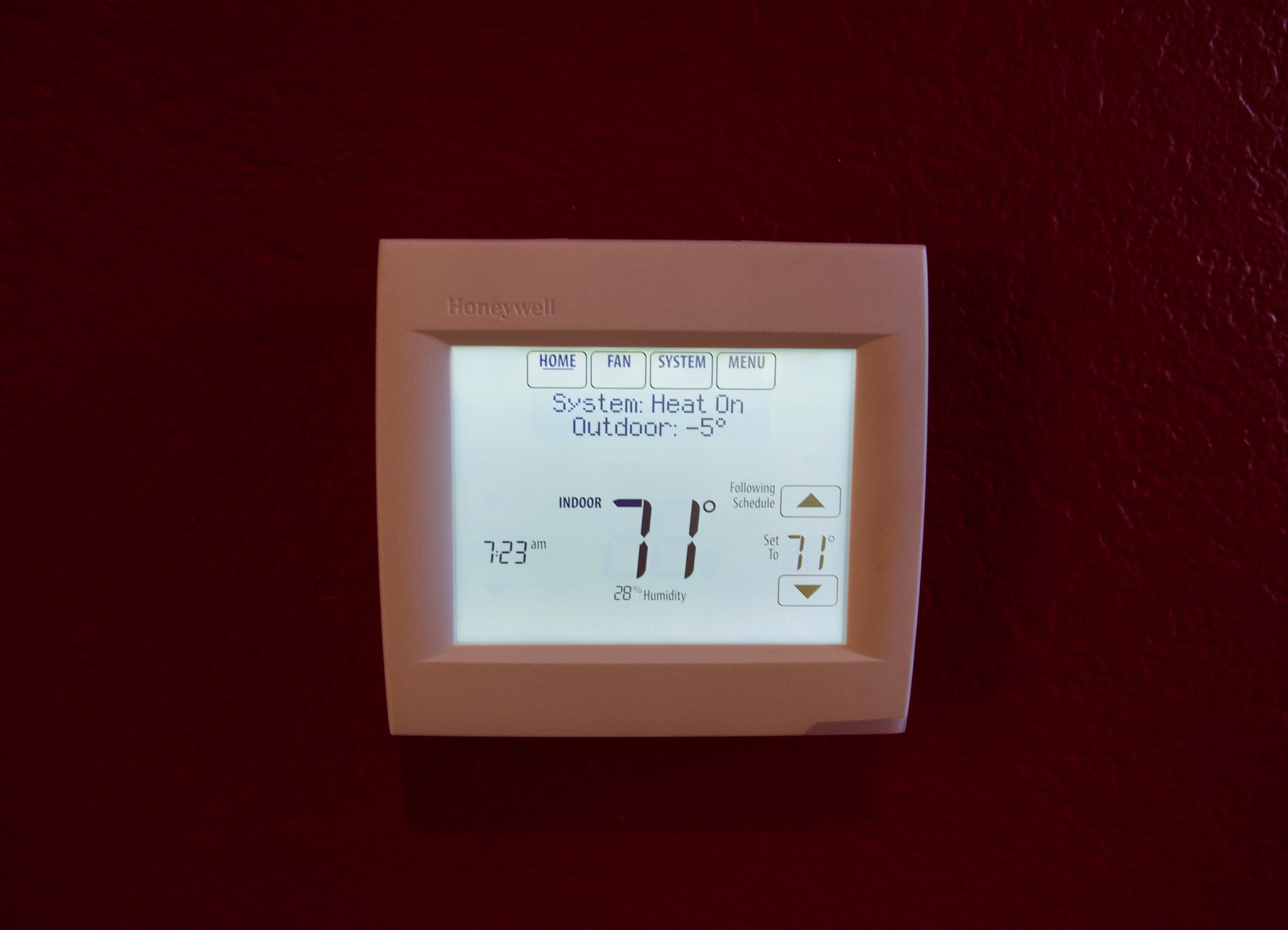The photograph is a slightly rectangular, landscape-mode close-up shot of a deep red, textured wall with a prominently featured electronic thermostat at the center. The thermostat, framed by a white border, displays the Honeywell logo in the top left corner. The device is square-shaped and features a detailed digital screen. At the top of the screen, from left to right, are four labeled boxes: "Home," "Fan," "System," and "Menu." Directly underneath is a line of text displaying "System," "Heat On," and "Outdoor," alongside a temperature reading of -5 degrees. Below that, on the left side, the screen indicates the current time as 7:23 AM. To the right of the time, the screen shows the indoor temperature of 71 degrees. On the far right, there is an adjustable switch with up and down arrows, set to 71 degrees and indicating "following schedule."